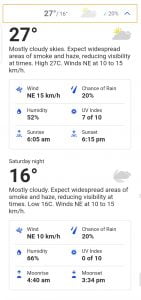A detailed weather report from a phone screen displays various weather statistics. The screen indicates a high temperature of 27°C and a low temperature of 16°C for the day. There's a 29% chance of rain, with mostly cloudy skies and widespread smoke and haze reducing visibility at times. Winds are noted to be coming from the east at 10 to 15 kilometers per hour. 

The display also includes a detailed chart summarizing these details. Additionally, it notes the sunrise at 6:05 AM and sunset at 6:15 PM. 

For Saturday night, the weather is mostly cloudy with widespread smoke and haze expected to reduce visibility. The low temperature is forecasted to be 16°C, and the winds are expected to be from the northeast at 10 to 15 kilometers per hour.

The chart comprehensively shows various icons and figures for wind speed, humidity, moonrise, moonset, and rain chances measured in inches, providing a complete overview of the day's weather conditions.